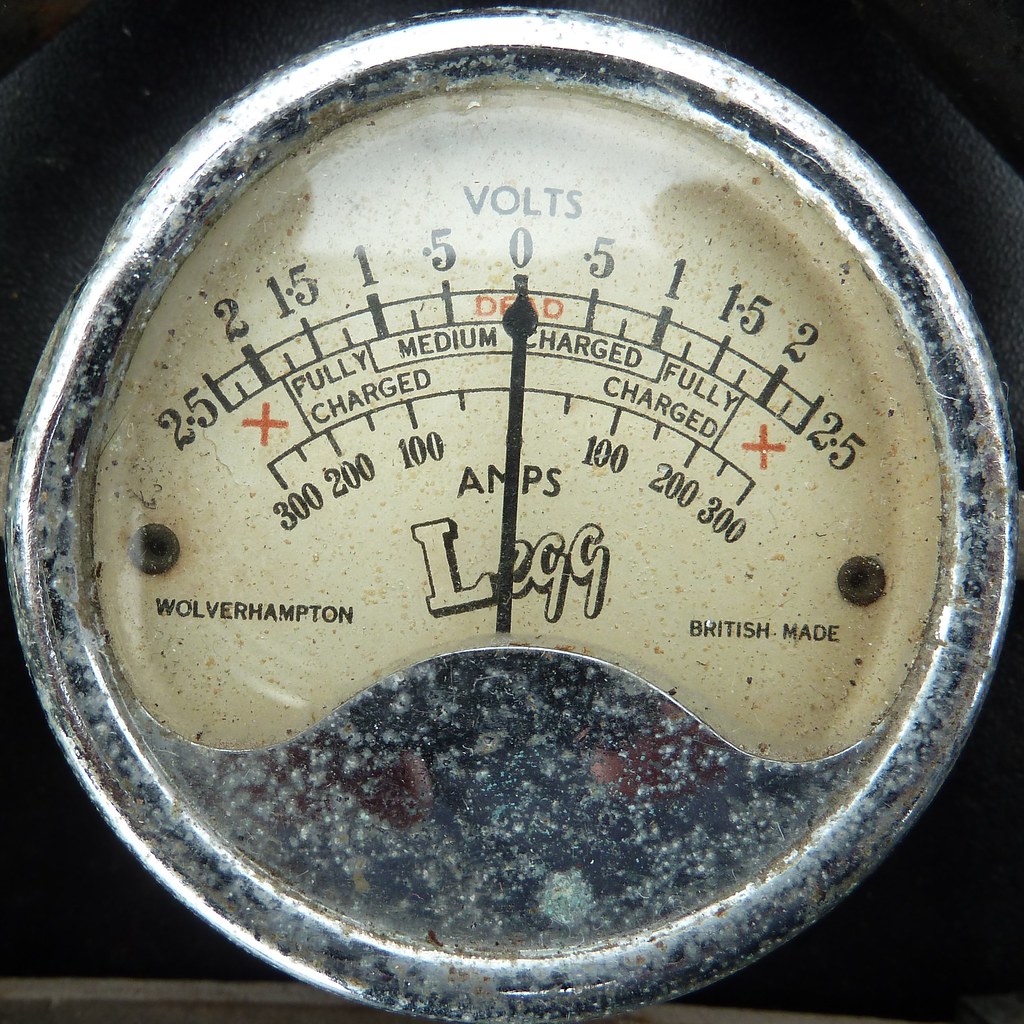The image is a close-up photograph of a very worn and weathered circular gauge, likely from an old piece of machinery such as a farm equipment or generator. The gauge is encased in a corroded and tarnished silver metal frame, indicative of prolonged outdoor exposure. The background behind the gauge is mostly black, with barely discernible shapes. The central dial is marked with an arm and pointer, currently indicating "0". At the top of the gauge, the word "VOLTS" is clearly visible. The scale on the gauge ranges from 2.5 on both ends, moving through increments of 2, 1.5, 1, 0.5, to 0 in the center, and then symmetrically back up to 2.5 on the other side. There are additional markings such as "fully charged" and "medium charged" with corresponding 'X' indicators. Beneath the scale, the word "AMPS" appears. The company logo "L.E.G.G." is centrally located on the gauge face. On the bottom left, the gauge reads "Wolverhampton," and on the bottom right, it states "British made." This detailed description points to the historical and utilitarian nature of the equipment, reflecting its likely age and robust use.